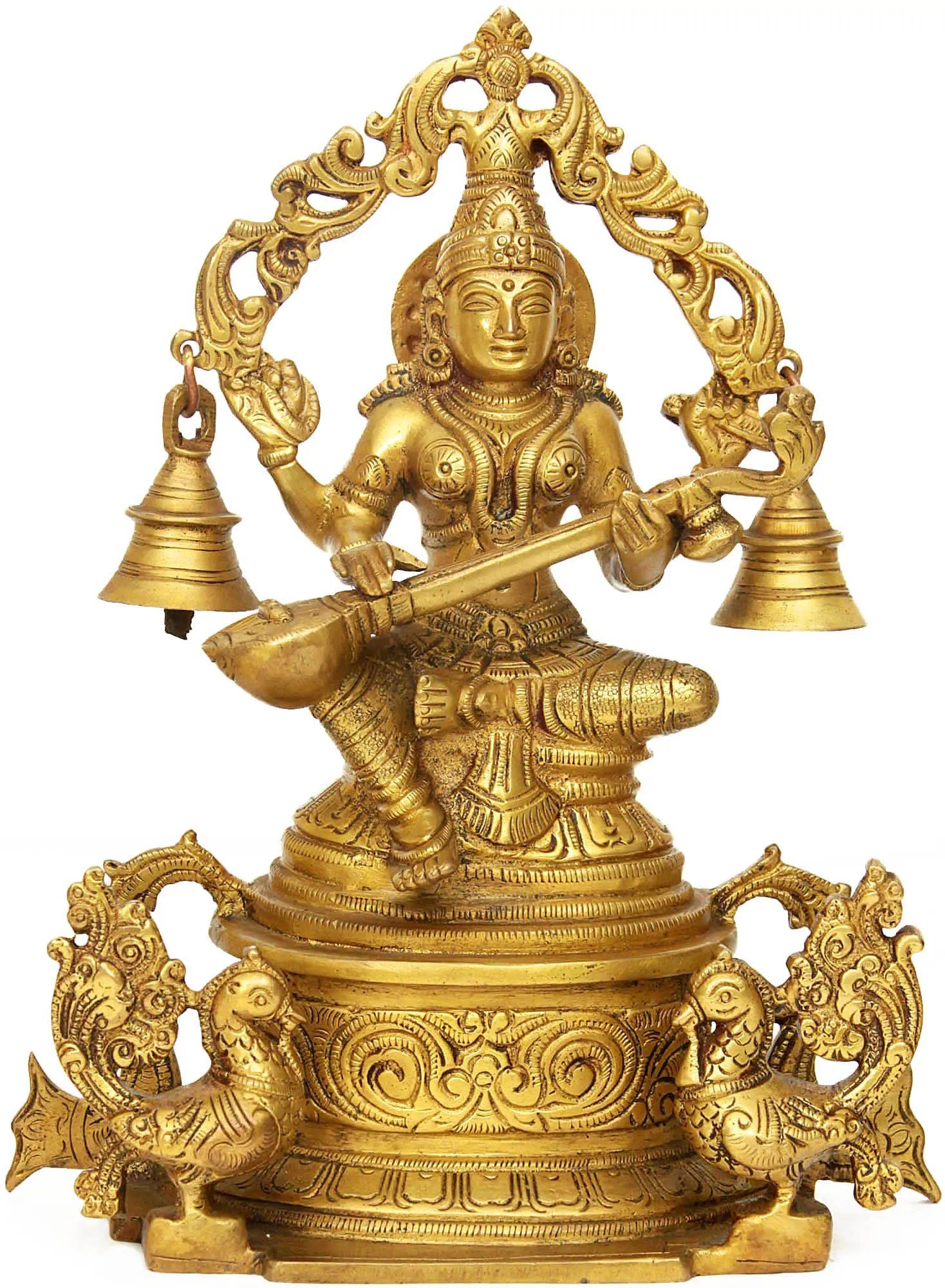The image features a golden-colored statue with an intricate design, placed against a stark white background. This elaborately detailed figurine, which could represent a Hindu deity, appears to be seated in a crisscross position atop a cushion or stand. The central figure, adorned in what seems to be traditional armor, has an array of arms—potentially four—each engaged in playing a musical instrument, emphasizing a sense of divine or celestial presence. The headpiece is notably ornate, with fleur-de-lis shapes extending outward, each adorned with a dangling bell at its tip. Additionally, there are multiple bells accentuating the entire figure, enhancing its intricate and ornate appearance. Flanking the deity are bird-like figures, possibly representing ducks, which extend along either side, adding to the statue's rich cultural symbolism and artistic detail.